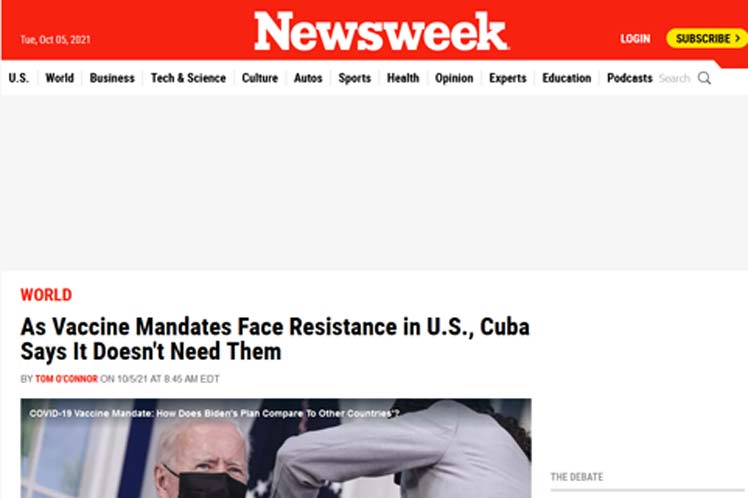The image depicts a Newsweek magazine layout. The left side features a white column with a red bar at the top. On this red bar, smaller print indicates the date as "TUE, OCT 05, 2021." Below the red bar, the large, bold text "Newsweek" is prominently displayed. On the right side of the image, there is an option to "Login" and a yellow oval-shaped "Subscribe" button with black text.

Directly below the top navigation bar, there are category links listed in bold black text separated by small lines, including "US," "Business," "Tech & Science," "Auto," "Sports," "Health," and "Opinion." Below these categories, a large gray bar spans the width of the image, occupying about half of the vertical space and remaining empty.

The lower half of the image highlights an article section. The section header "WORLD" is written in red capital letters. The title of the article is prominently displayed in larger black bold text: "As Vaccine Mandates Face Resistance in US, Cuba Says It Doesn’t Need Them." The byline follows, with the author’s name, "Tom O'Connor," in bold red letters, and the date and time, "10/05/21 at 8:45 AM EDT," in smaller black text.

Below the article headline, an image of Joe Biden receiving a COVID-19 vaccine is situated, showing only his head and the arm of the healthcare worker administering the shot. Accompanying the image, a caption reads: "COVID-19 Vaccine Mandate: How Does Biden's Plan Compare to Other Countries?"